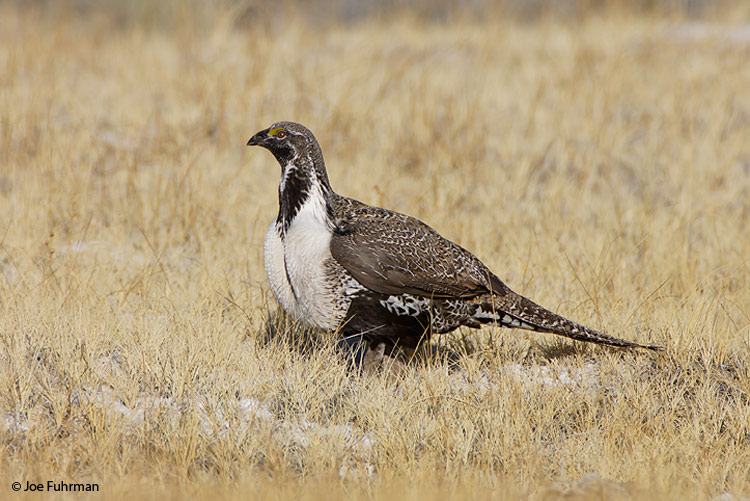In this outdoor photograph, a bird stands poised in a field of tan, dead grass that gives the scene its distinct hay-like appearance. The light-colored ground, intermittently dotted with small patches of snow, suggests a wintry landscape. The bird, likely a grouse based on its features, is positioned centrally, offering a close, zoomed-in view that highlights its distinct plumage.

The avian subject boasts a striking combination of colors: a white breast contrasts with dark, chocolatey brown feathers adorning its wings, long tail, and small, puffy head. The head itself is a blackish-brown hue, and the bird's beak is entirely black. Notably, the eyes are encircled with a yellowish tint, giving the bird a piercing gaze. Despite its large size, comparable to a slightly elongated chicken, the feet remain obscured by the dense grass.

In the lower left corner of the image, the photographer's credit, "© Joe Furman," is visible, ensuring proper attribution. The detailed and vivid depiction captures the essence of the scene, merging the stark natural beauty of the bird with the subtly wintry environment.